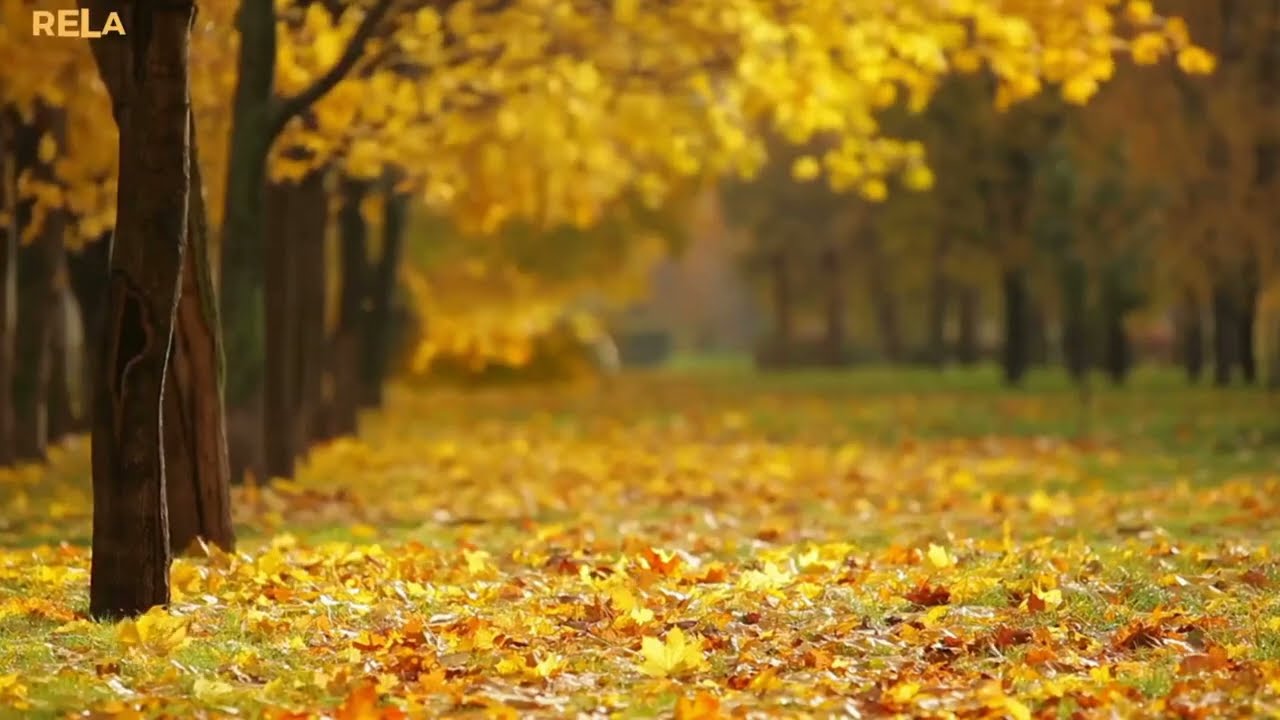The image depicts a serene outdoor autumn scene in a forested area, characterized by meticulously aligned rows of dark brown barked trees on the left side, extending into the distance where they become indistinct and blurry. The trunks are topped with branches adorned with bright yellow leaves that stretch across the image, creating a radiant golden canopy. The ground below is a vibrant carpet of fallen leaves in varying hues of yellow, orange, and red, interspersed with patches of green grass. Additional trees populate the background on the right, their leaves a mix of green, red, and yellow, though they appear less distinct due to the distance. Prominently situated in the upper left-hand corner is a four-letter word, "RELA," enhancing the photographic composition. The foreground showcases the sharpest details, particularly the fallen leaves, while the background remains softly out of focus, emphasizing the depth and tranquility of this autumnal tableau.